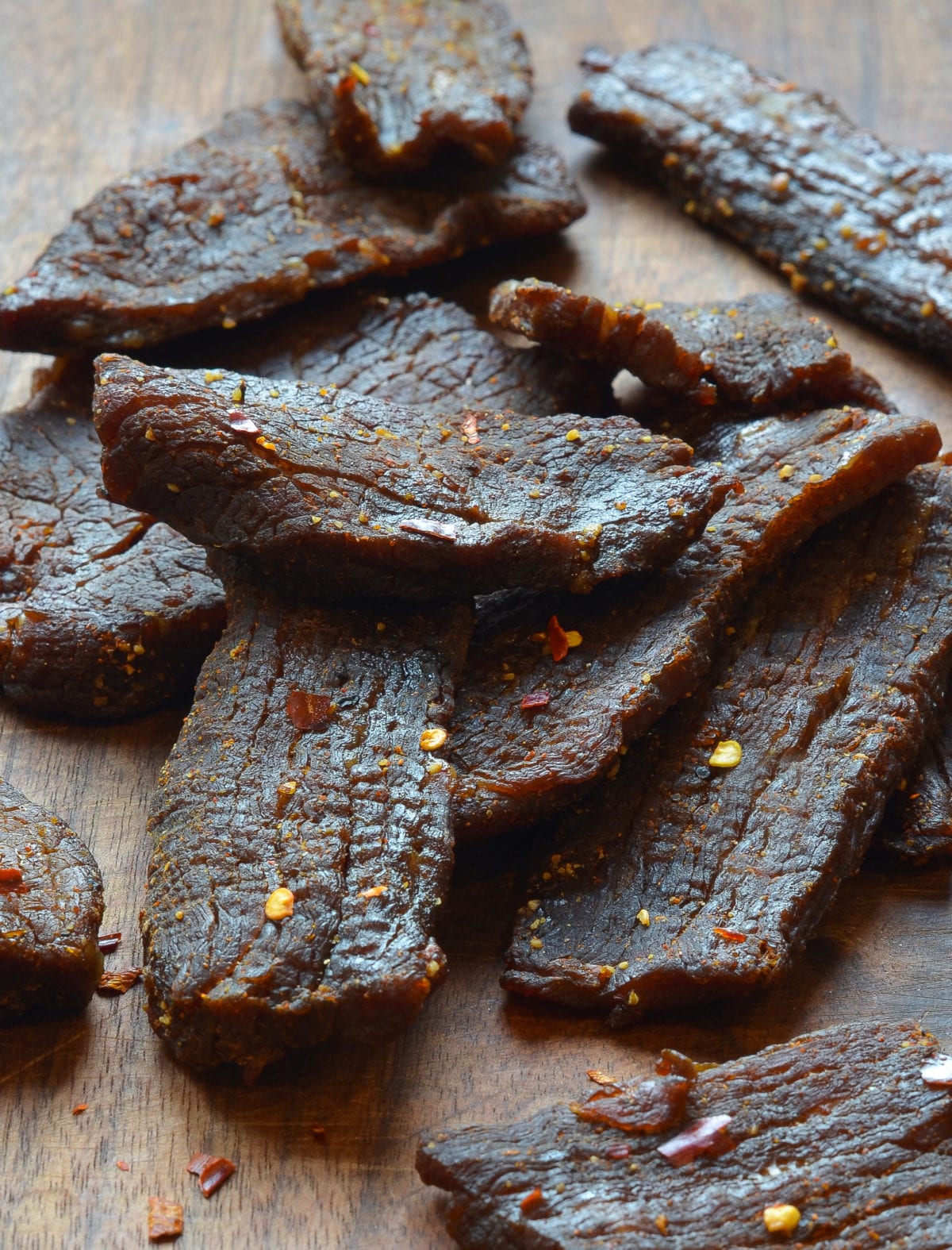This close-up photograph captures a pile of approximately 12 to 15 pieces of beef jerky arranged on a finished wooden table. The jerky pieces, varying in hues from deep brown to reddish, are sprinkled generously with small red and yellow pepper flakes, adding a spicy visual texture to the scene. Some pieces of jerky are curled over, hinting at their thickness—about a quarter inch—and length, roughly two to three inches. The natural lighting emphasizes the details, making the pieces in the foreground sharply focused while those in the background appear slightly out of focus. No text is present to specify the exact type of meat, but the overall composition and intricate detailing suggest a fresh, flavorful variety of beef jerky.